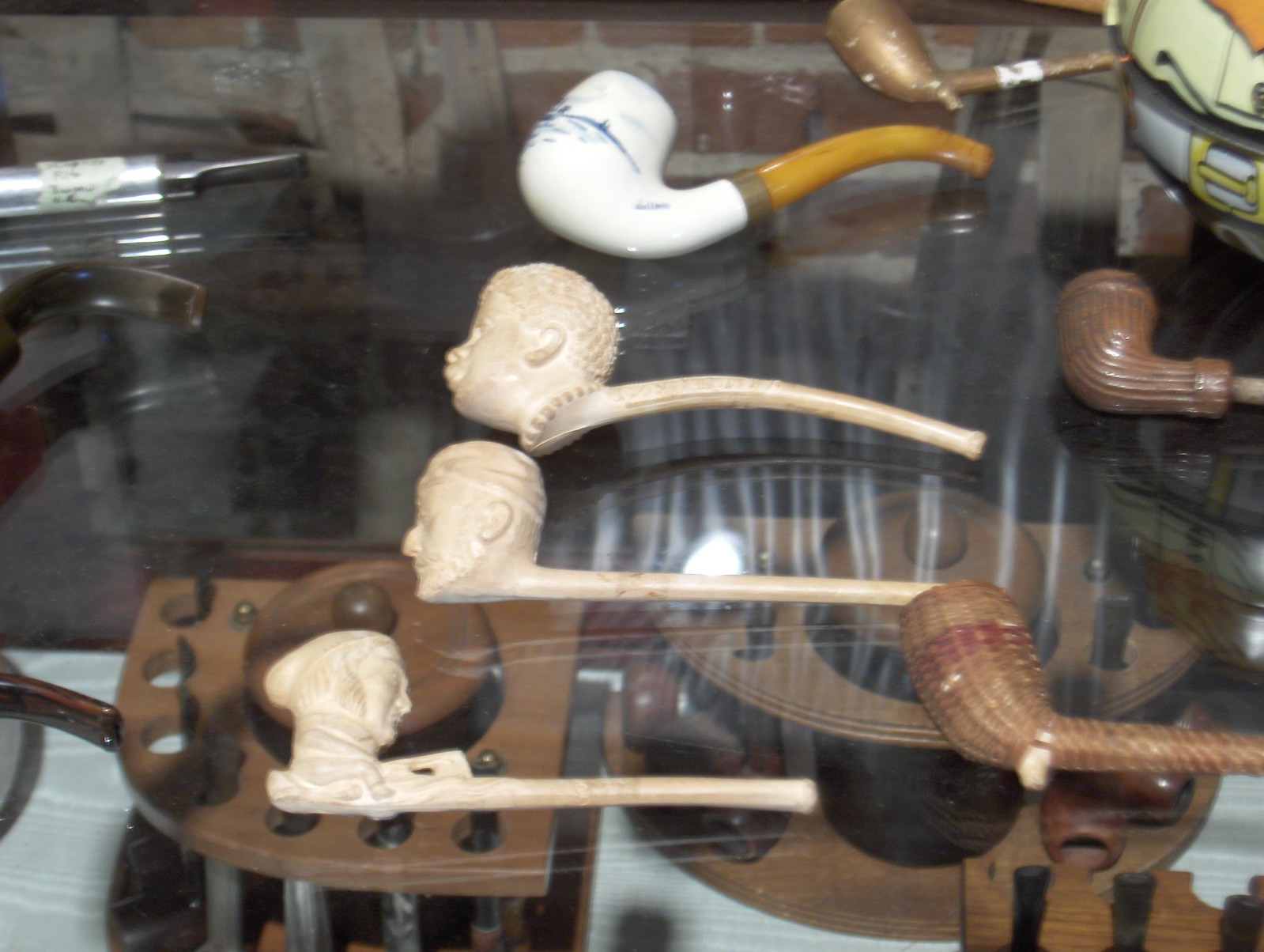This detailed photograph captures a collection of seven intricately designed smoking pipes displayed atop a glass tabletop, with a brick wall faintly visible in the background. Central to the display are three tan-colored pipes, each with a bowl intricately carved to resemble human heads, featuring detailed depictions of textured hair, facial features, and ears. These pipes each extend into long mouthpieces, with one being notably curved while the others are straight. Additionally, a glossy white ceramic pipe with a light yellow mouthpiece stands out, adorned with a dark blue or black decorative pattern on its front. There is also a pipe that appears woven like a wicker basket, another brown pipe, possibly made to mimic the appearance of cane, and a complex white pipe featuring a head that resembles a historical figure from George Washington’s era. Completing the collection are two distinct pipes - one with a striped brown end and grooves, and another sizable one with a white bowl accented with blue patterns, transitioning into a brown mouthpiece with a golden hue tip. Scattered behind the pipes are some indeterminate white and yellow objects, providing additional depth to the display case's contents.